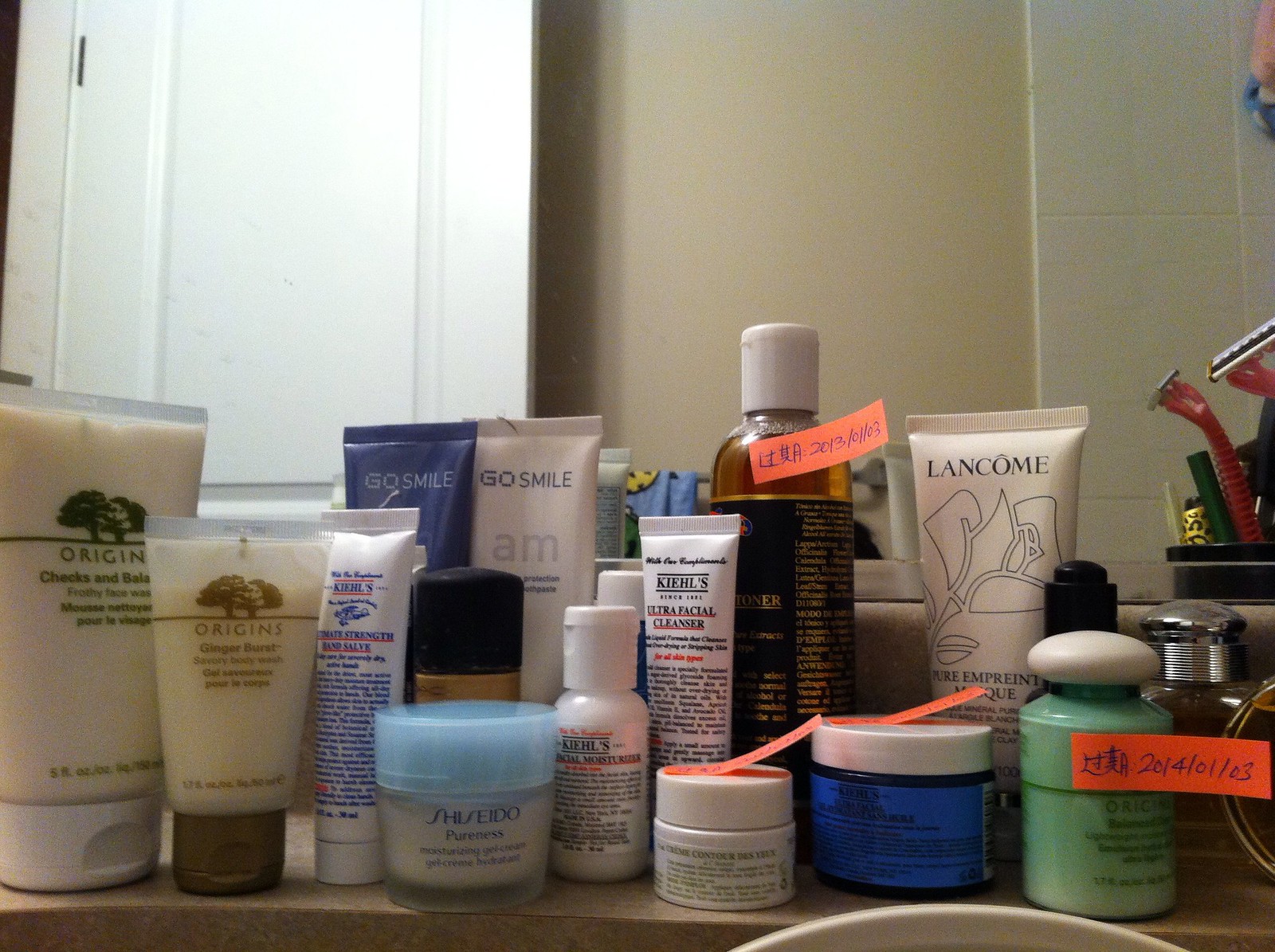The image depicts a cluttered bathroom vanity laden with a diverse assortment of toiletries and self-care products. Prominently positioned on the surface are two tubes from the Origins skincare line, featuring distinct labels with illustrations of large trees—one with green trees and lettering and the other with brown trees and lettering. The tubes stand inverted on their caps for easy access. Interspersed among them are small tubes of various brands, including Go Smile and Lancome.

On the right side of the vanity, a green bottle with a white cap sits adjacent to a squat, blue bottle, also with a white cap. The rightmost edge of the image reveals a holder containing several razors with plastic handles. The backdrop consists of a tiled wall to the right and a white door to the left, opening inward to the bathroom.

The image appears to be taken from the perspective of a reflection captured in a mirror behind the vanity. This mirror also reflects a light tan wall at the center, providing a glimpse into the surrounding bathroom environment. The entire scene is an intricate display of everyday self-care essentials arranged in a seemingly haphazard manner.